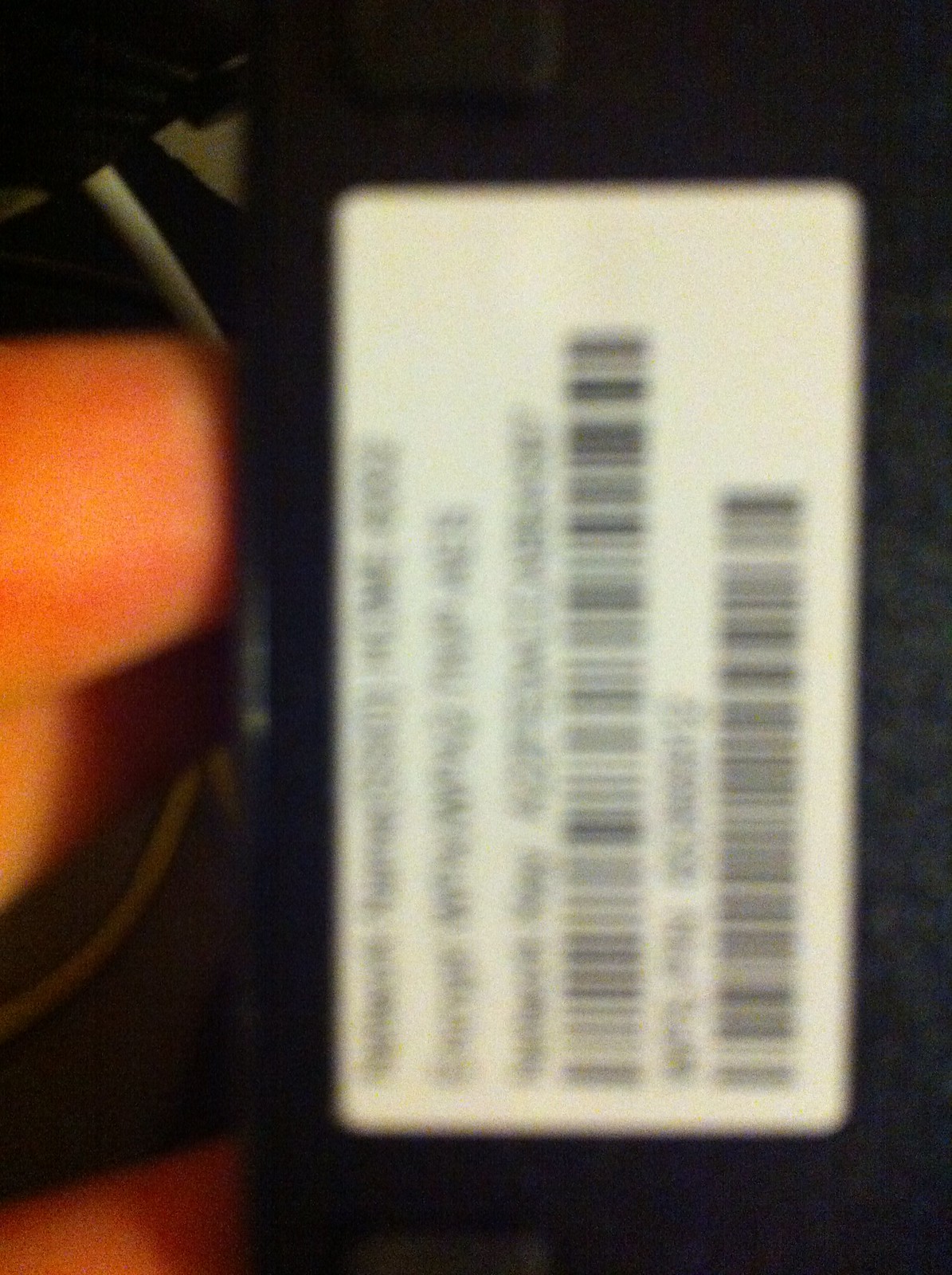This photograph is significantly blurred, obscuring many details. On the left side of the image, the blurry outlines and shading suggest the presence of a person's fingers, indicating someone might be holding the object in the scene. Dominating the right side of the picture is a large, black object. A prominent rectangular white label is affixed to this object. The label features two barcodes at the bottom, above which are some numbers that are indistinguishable due to the blur. There is a line of text above the barcodes, providing a description that remains unreadable in the photograph. Additionally, the upper-left corner of the image shows a material with a shiny texture, possibly forming part of a base connected to the black object, adding to the intrigue of the photograph's contents.